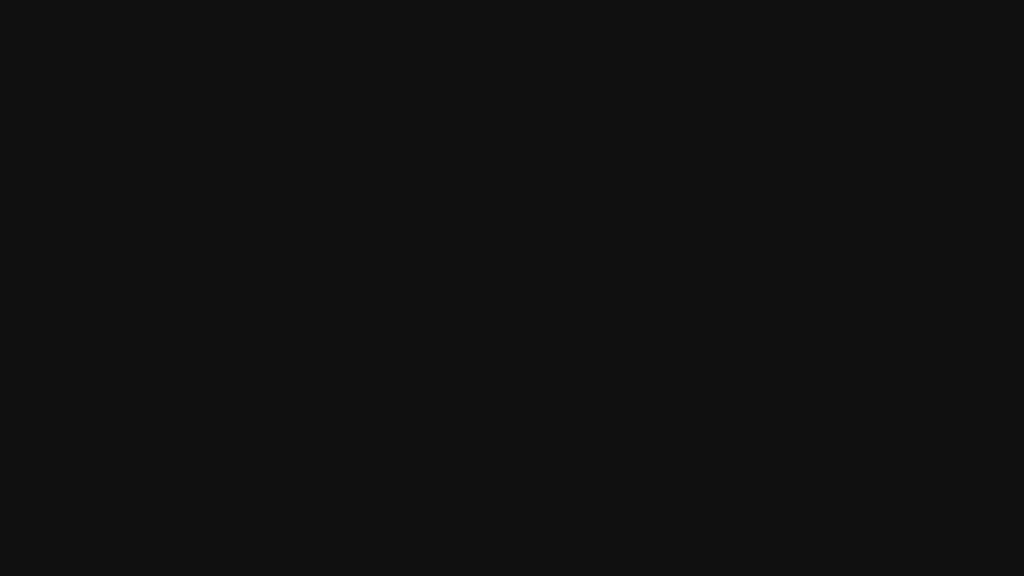This image features a rectangular black box occupying the entire frame. The box is exceptionally wide and both its length and height create a perfect rectangle, generating a sense of uniformity. The background within the box is a deep, uninterrupted black, devoid of any text, photos, links, lines, or buttons. The plain black background dominates the image, making it appear as a large, featureless, and perfectly rectangular shape. The simplicity of the composition ensures that no other visual elements distract from the stark blackness of the box.